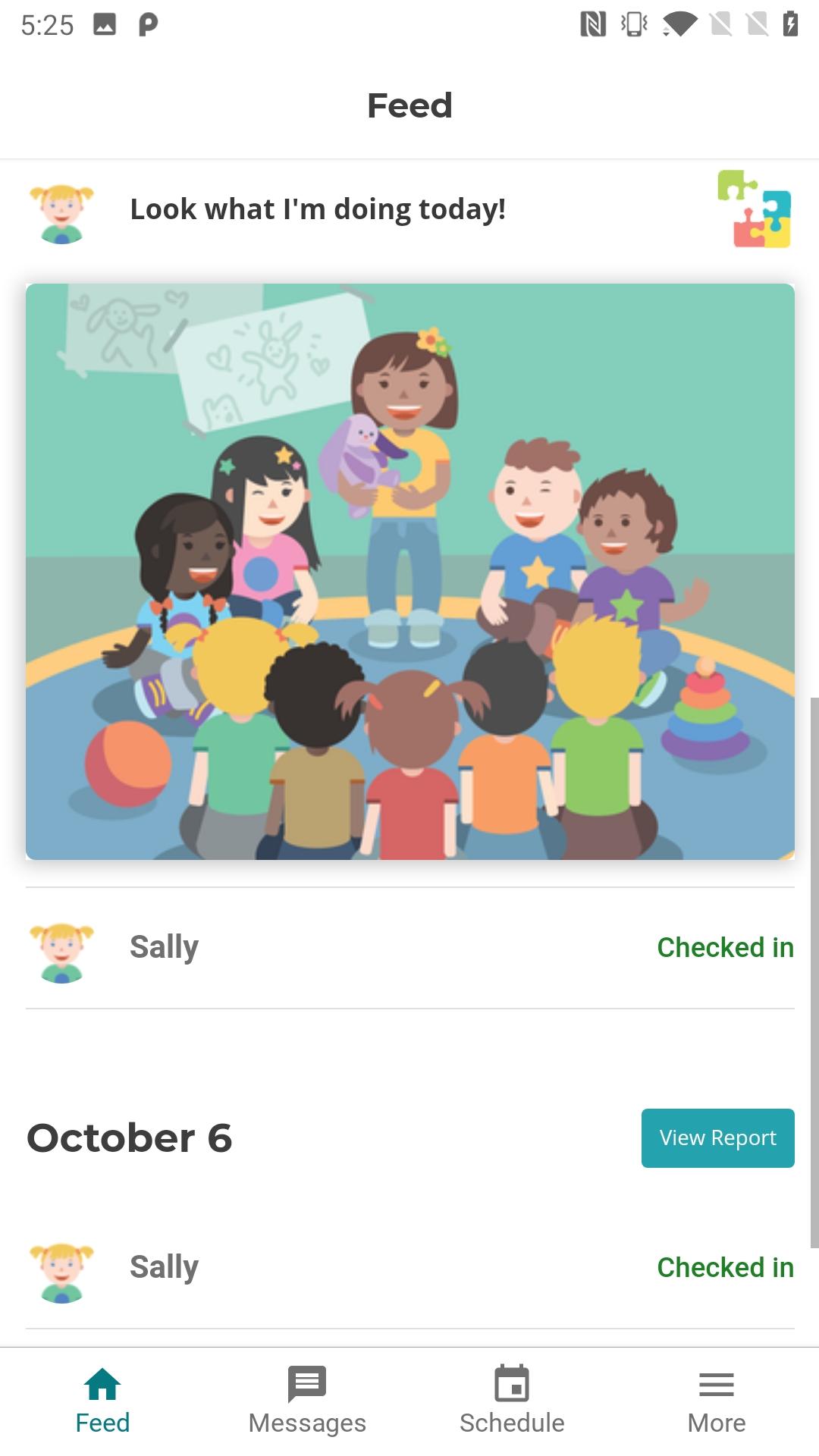A screenshot of a children's app is displayed, showcasing a feature titled "Feed." The feed highlights a post captioned "Look what I'm doing today," featuring an image of a vibrant and diverse classroom filled with cartoon-like characters. In the image, a group of children are sitting in a circle, engaged in playful activities. The scene is diverse, with children of various ethnic backgrounds—Black, White, Asian—interacting together. A girl named Sally has the label "checked in" next to her name, signifying her presence or participation in the app's activities.

At the center of the image, one girl stands holding a stuffed animal, radiating joy as she smiles brightly. The other children around her are likewise happy, either smiling or laughing. Scattered among them are a few toys, including a ball on the left and a colorful ring-stacking toy, adding to the cheerful atmosphere. The app appears to be designed for monitoring and engaging children's activities, allowing users to keep track of daily interactions and participation within a fun, communal setting.